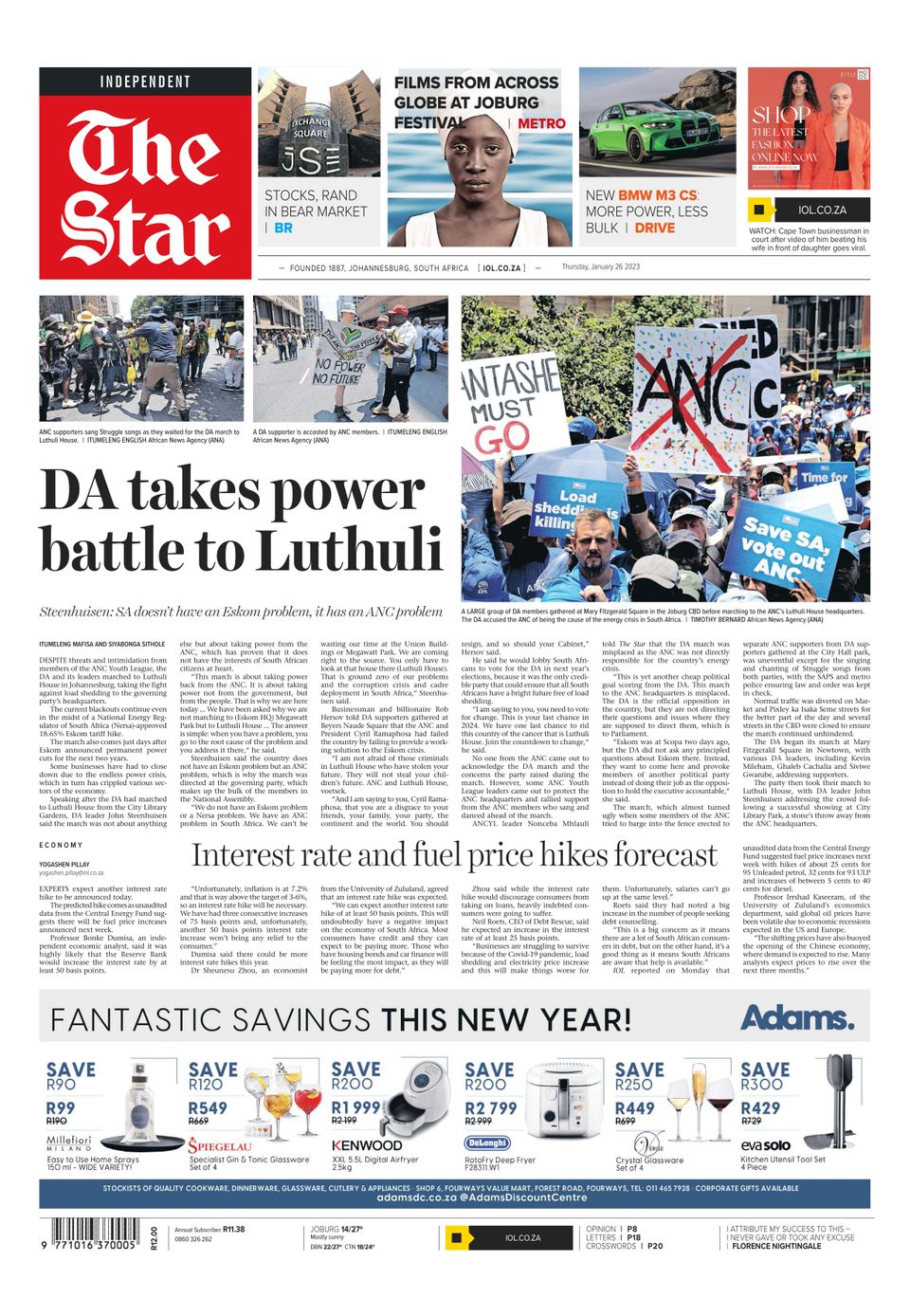The screenshot showcases a collage of various images and headlines, each occupying distinct sections. In the top left corner, a black bar labeled "Independent" spans across, accented by a red rectangle with "The Star" boldly written in large white text. Adjacent is a collection of magazine covers featuring diverse subjects. Prominently, an African American woman is seen wearing a white turban and a white toga. To her right, a sleek, dark green sports car is displayed. Below, a group of models clad in striking orange leather jackets and pants are featured.

A bold black headline on the left reads, "DA takes power battle to Luthuli", alongside an image of protesters brandishing colorful signs. One sign, resembling graffiti art in blue, red, and yellow, is marked with a large red X over black letters "A" and "C". Another sub-headline announces, "Interest rate and fuel price hike forecast."

Towards the bottom right, a dark gray rectangle with black text heralds "Fantastic Savings," with the phrase, "This New Year!" emphasized in bold. To its immediate right, "Adams" is written in dark blue. The far right of the image features an assortment of wine glasses and bottles, suggestive of a wine selection display.